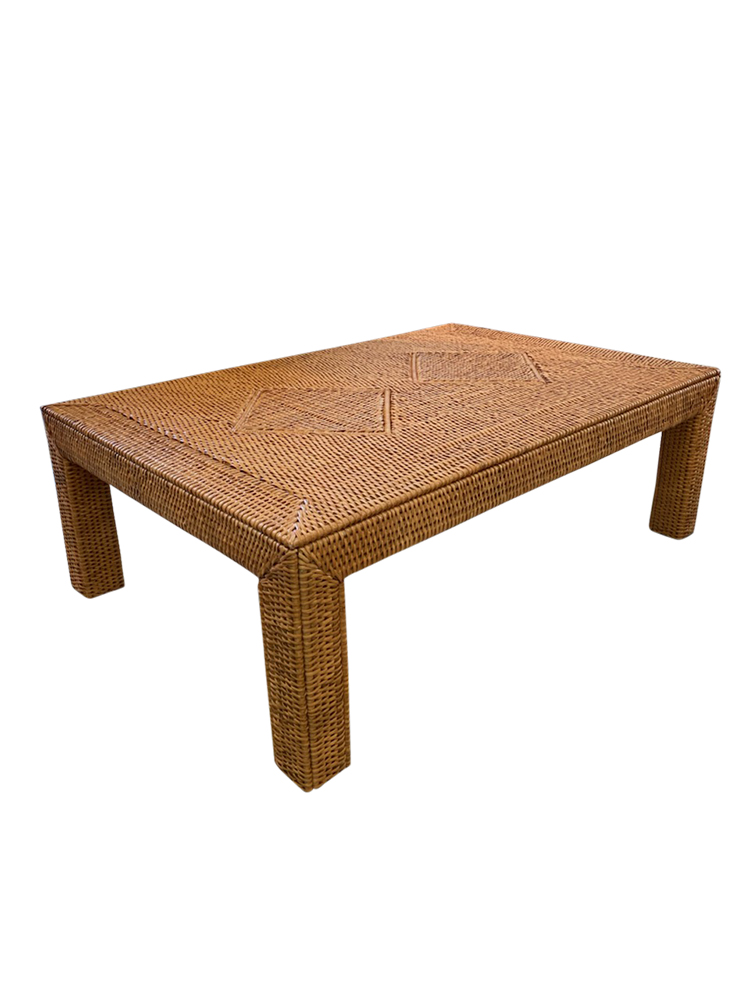The image depicts a small rectangular table or footstool, woven intricately from a wicker-like material with a light to dark brown color palette, exuding a glossy, golden-brown hue. The entire surface and four legs of the table display a fine, consistent weave pattern, giving it a textured appearance. Prominently placed in the center of the top surface are two large, woven diamond shapes, bordered by distinct lines that set them apart from the rest of the weave. The table is viewed from an angle, showing three of its four legs clearly, with the fourth leg obscured. It sits against a plain white background, emphasizing its detailed and artisanal construction.